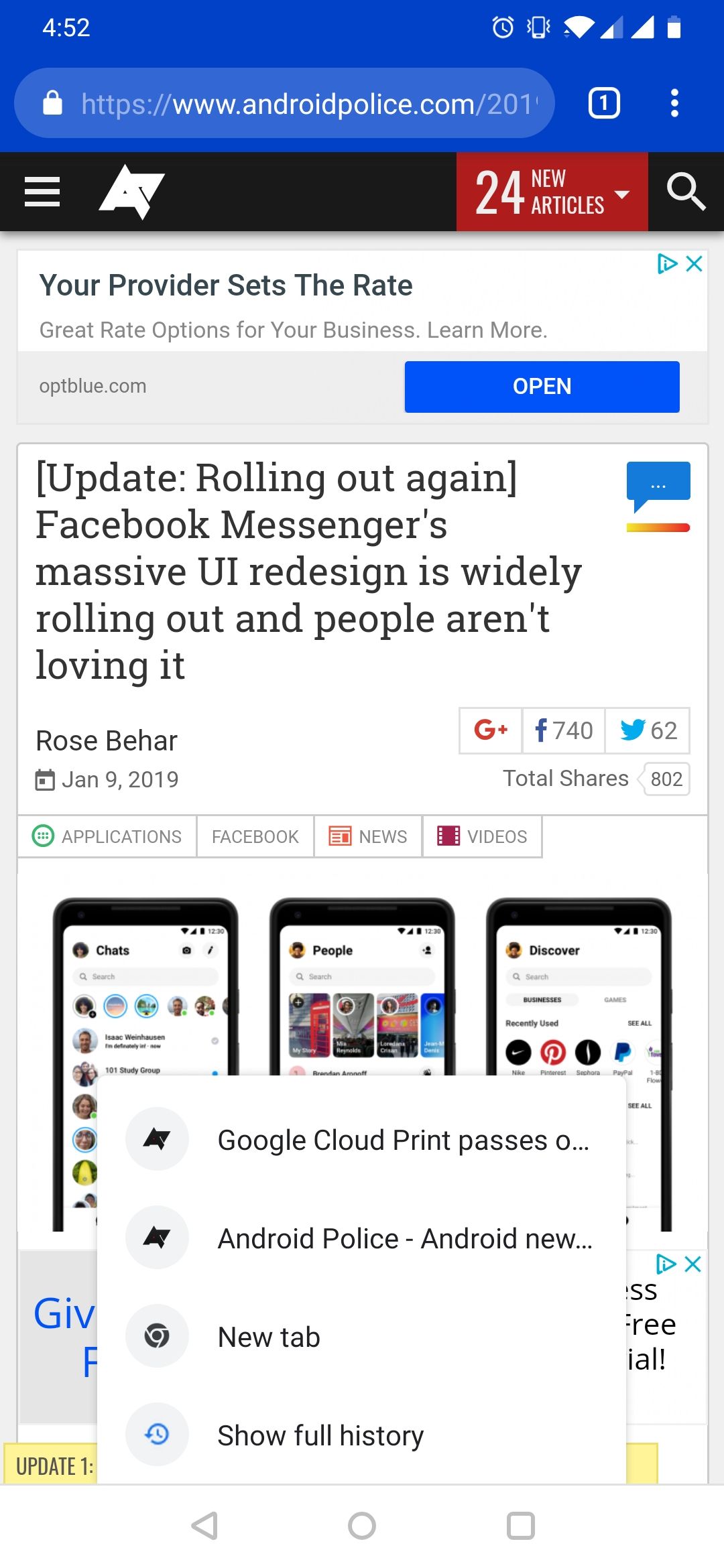The image depicts a smartphone displaying a search for "androidpolice.com" on its screen. The top of the phone screen is blue with white lighting, and the time displayed is 4:52 PM. The device shows various status icons including an alarm, cellular signal bars, Wi-Fi signal bars, and a battery indicator. Below the status bar, there's a black band featuring a hamburger menu (three stacked lines) on the left side and a notification badge indicating "24 new articles" in red with white text.

The main content of the screen includes a banner ad with the text, "Your provider sets the rate, great rate options for your business. Learn more. Open" in blue, with a mention of "optblue.com." Below the ad, there is a headline stating "Update rolling out again: Facebook Messenger's massive UI redesign is wildly rolling out, and people aren’t loving it," authored by Rose Behar on January 9th, 2019, with total shares amounting to 802.

Additionally, there is a section labeled "Applications" listing Facebook news and videos. Underneath this section, there are images of three smartphones displaying different charts or chats. At the top of each phone image, the word "Discover" is visible. Above the phones, a white horizontal rectangle contains the text "Google Cloud Print Passes, Android Police, Android New, and New Tab." The caption mentions options to "Show full history."